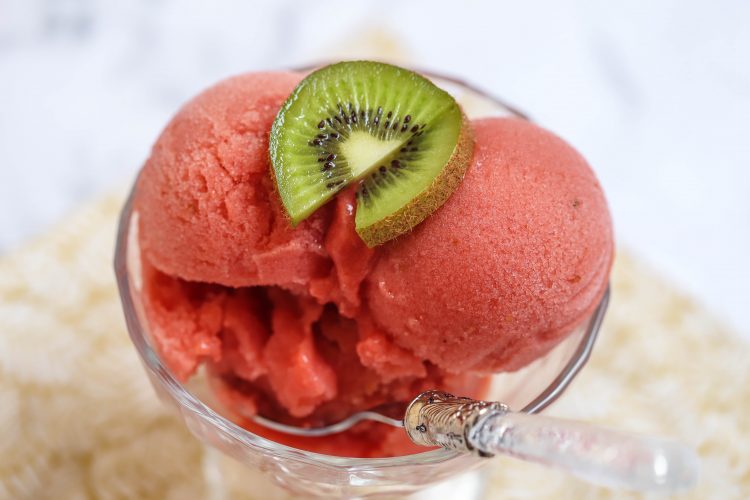This horizontally aligned, landscape-oriented photograph centers around a close-up of a frozen dessert in a clear glass bowl. Positioned in the glass bowl are two reddish-pink scoops of what appears to be raspberry sherbet or a tropical-flavored ice cream. The ice cream scoops slightly overflow the edges of the bowl. A decorative spoon with a see-through handle and a gold middle part, or possibly a silver shank, emerges from the lower right corner and extends beneath the ice cream. Atop the dessert sits a single round slice of kiwi with a triangular notch cut from its edge. The background is softly blurred with bright, oversaturated lighting, featuring a mostly white and beige marble-like surface.